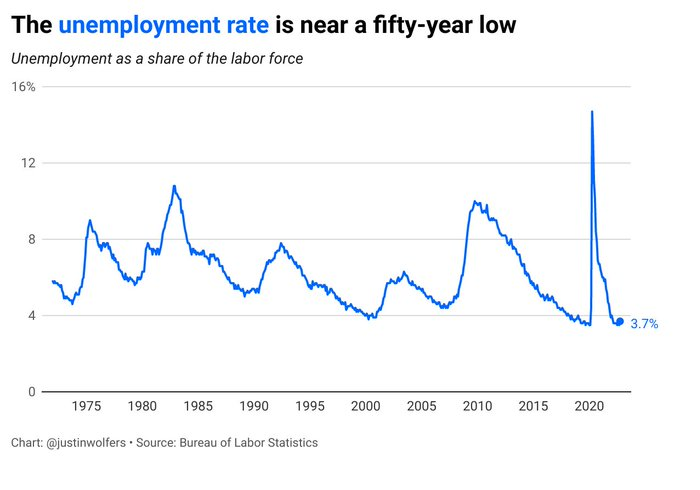The image features a detailed graph depicting the unemployment rate as a share of the labor force from 1975 to 2020, set against a white background. The x-axis represents the years, marked at intervals from 1975 to 2020, while the y-axis shows unemployment percentages, ranging from 0% to 16%. A blue line meanders across the graph, illustrating fluctuations in the unemployment rate over the years. The graph begins at approximately 5.5% in 1975, peaks near 10% in 1982-1983, and decreases to around 4% in 2000. Another rise occurs around 2010, reaching 9%, with the highest peak near 14% in 2020 during the pandemic, before finally dropping to about 3.7%. Above the graph, the title reads, "The unemployment rate is nearly a 50-year low," followed by a subheading, "Unemployment as a share of the labor force," with "unemployment rate" highlighted in blue. At the bottom, the graph cites its source as the Bureau of Labor Statistics, with credit given to Justin Wolfer.